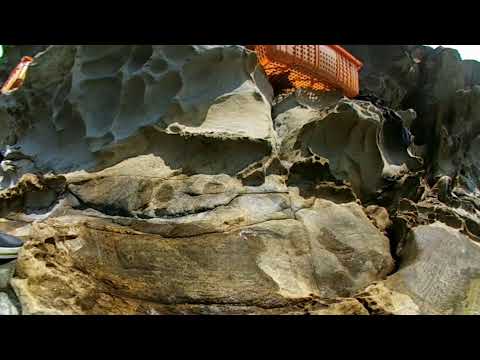The image depicts a rugged mountainous ridge littered with a multitude of large, jagged rocks of various shapes and sizes. The rocks predominantly display a silver-gray color with occasional rusty brown hues. Towards the middle-top section of the image, resting among the rocky outcrops, is an orange structure resembling an observation deck or basket, likely intended for tourists to enjoy panoramic views of the surrounding valley. The deck stands out against the monotone landscape, which otherwise lacks any signs of human or animal presence. In the bottom left corner, a glimpse of a navy blue and white shoe is visible, hinting at a human footprint in the otherwise desolate, rocky terrain. Additionally, near the bottom right, there is a large dark rock with a shadowed area that might be a cave entrance, adding a mysterious element to the scene.